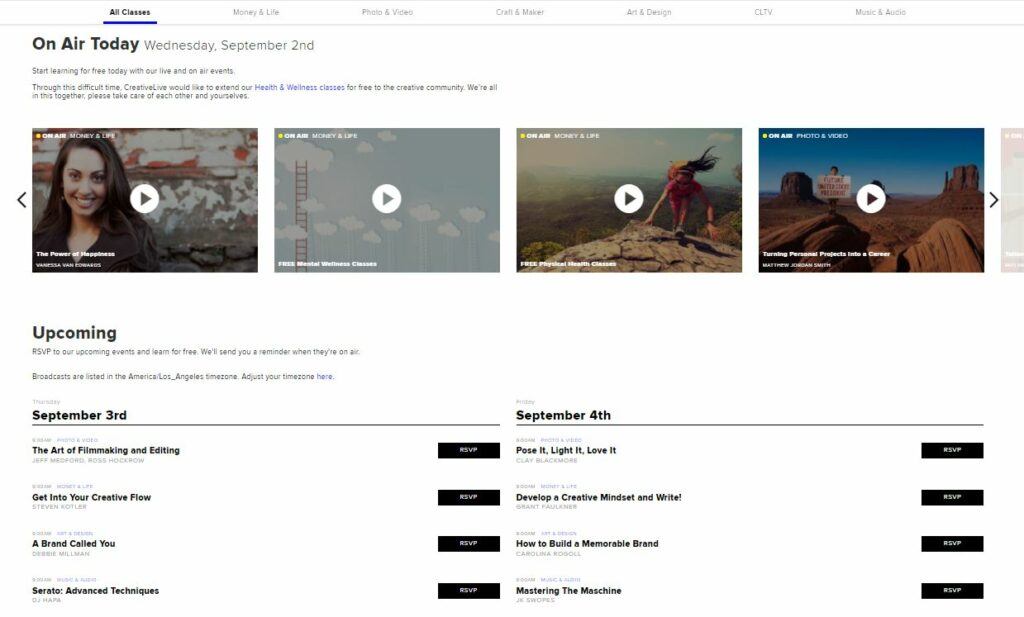This is a rectangular image oriented horizontally. Across the top, a white banner spans from left to right, bordered by two thin gray lines. The banner features a menu with a series of categories. The first menu option, labeled "All Classes," is underlined with a purple line and written in bold dark black font. The remaining menu options appear lighter and include "Money and Life," "Photo and Video," "Art and Design," and "CUN." One category remains unreadable.

Beneath this menu, the heading states "On Air Today, Wednesday, September 2nd," followed by text that is too small to discern. Below this description, there are four clickable thumbnail images, each marked with a white circle containing a black play triangle, suggesting they are video previews. 

1. The first thumbnail features a woman smiling directly at the camera with an outdoor wall background.
2. The second thumbnail shows a cloudy sky with a ladder extending upwards on the left side.
3. The third thumbnail depicts someone standing atop a rock they appear to have climbed.
4. The fourth thumbnail appears to show a desert landscape.

Below these thumbnails, the heading "Upcoming" is displayed, with additional text beneath it mentioning events on "September 3rd and 4th."